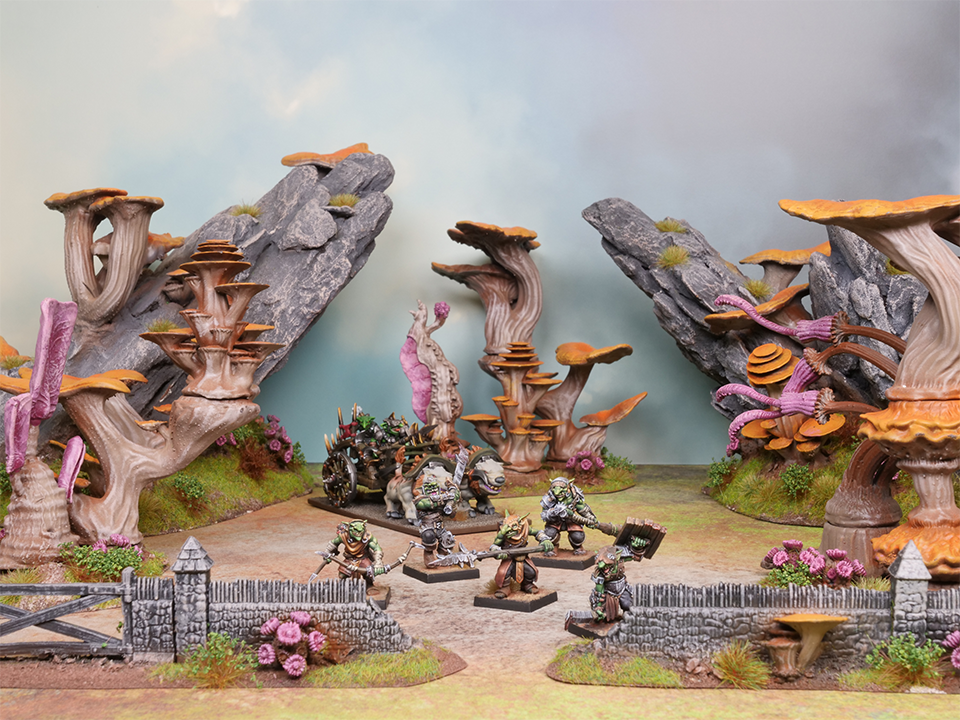In the image, a meticulously arranged scene of Dungeons & Dragons (D&D) miniatures is displayed, featuring a vibrant and colorful fantasy environment. The backdrop is a light blue cardboard sky, which sets the stage for the detailed setup. On both sides of the scene, there are tall rock formations and tree-like structures whose tall trunks are topped with large, mushroom-esque caps in shades of yellowy brown, pink, orange, and purple.

In the foreground, stone fences frame the display, creating a boundary for the action within. The ground is dotted with green bushes and grass interspersed with pink flowers, adding to the visual richness. At the center, a variety of intricately painted figurines, likely pewter, are strategically positioned. Among them are characters resembling bears and armored monsters wielding weapons such as bows, swords, and warhammers. Additionally, a chariot, pulled by whimsical, one-eyed, four-legged beasts, adds to the imaginative scene.

Overall, the arrangement exudes a sense of vibrant activity and fantasy, with its colorful elements and carefully positioned miniatures suggesting a moment captured from an epic tabletop battle, possibly staged for a toy catalog or a photographic showcase.